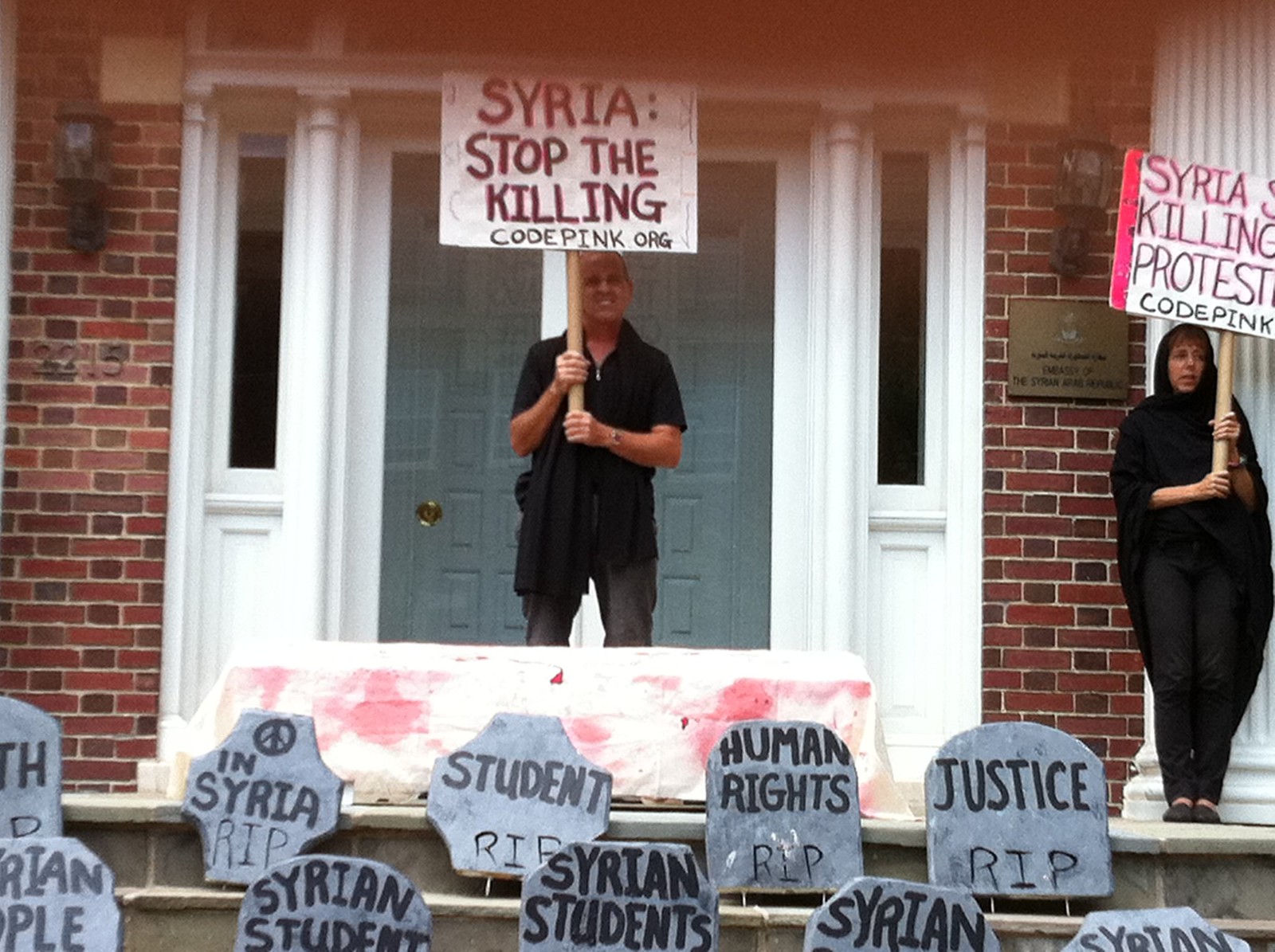The image depicts a protest scene in front of a brick building with white columns and a large white door. Two individuals are prominently featured on the top step: a man in a black short-sleeved collared shirt and black slacks, and a woman in a black hijab and black clothing. The man is holding a large sign with reddish-black letters on a white background that reads, "Syria: Stop the Killing, CodePink.org." The woman’s sign also references Syria, stopping the killing, and CodePink, though part of the text is cut off in the image. 

At the base of the steps are makeshift gravestones, painted gray with black lettering, bearing messages like "R.I.P. students," "R.I.P. human rights," "R.I.P. justice," and "R.I.P. Syrian students," symbolizing the losses in Syria. The building has a bronze plaque, suggesting it may be a public institution. The overall scene powerfully highlights the protest against the violence in Syria, organized by CodePink.org, with symbolic gravestones underscoring the gravity of the situation.